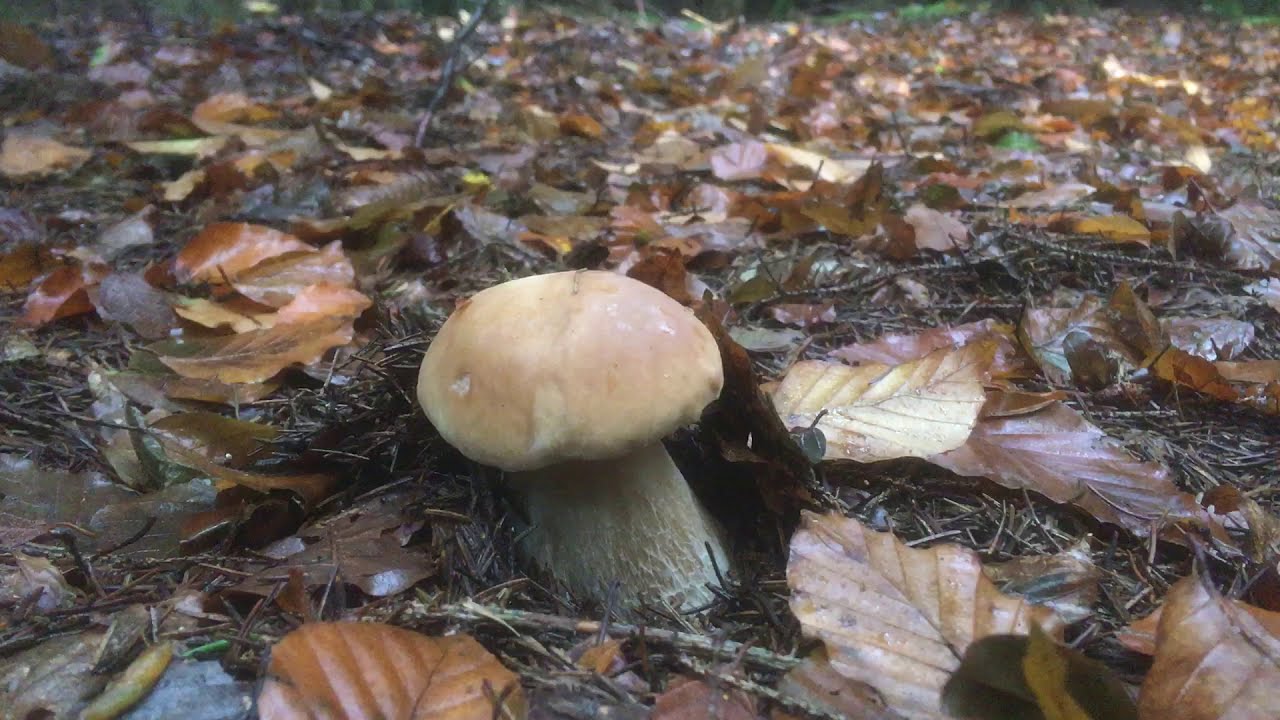The photograph captures a serene, damp forest floor, laden with a thick layer of brown, dried leaves that glisten with recent rainfall. At the center of this autumnal scene stands a large mushroom, its thick, gray stem supporting a wide, light brown cap. The mushroom's meaty texture contrasts vividly against the dense carpet of wet leaves and scattered twigs, hinting at the forest's coniferous nature with needles sporadically visible amongst the foliage. In the background, the leaf-strewn ground stretches into the depths of the forest, devoid of any people or animals, encapsulating a moment of quiet solitude and natural beauty.